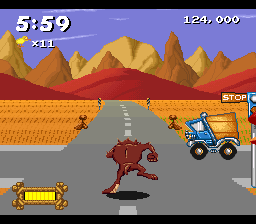A vibrant scene from a retro 16-bit video game, reminiscent of the Nintendo or Super Nintendo era, featuring an active gameplay moment. The central character, possibly a bear or a creature akin to the Tasmanian Devil, is depicted with a slender build, a bulky chest, and smaller limbs, sprinting down a grey highway with broken white stripes. The character appears to be disregarding a stop sign, just as a small blue truck with an orange cab and trailer approaches. This action takes place in a desert setting, with expanses of sand lining the road and distant brown and red mountains piercing the sky. A health bar, located in the bottom left corner, indicates full health, while the top right corner displays an impressive score of 124,000 points. A timer counting down from 5:59 and an icon showing the player has 11 lives left are also visible, adding to the urgency and dynamic action captured in this moment.